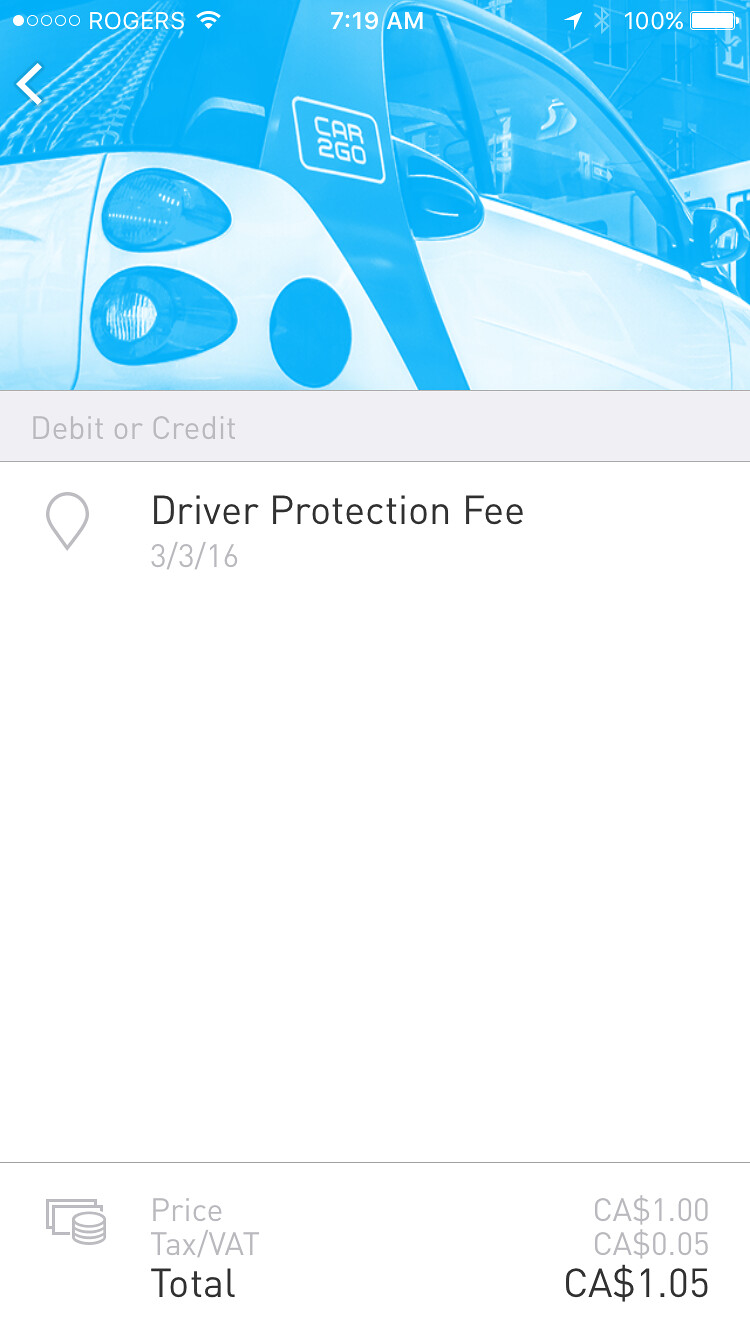The screenshot from a mobile phone displays an app interface related to automotive services. The top section shows the time as 7:19 AM, a full battery at 100%, and a Wi-Fi connection. A graphic of a car in blue, green, black, and white is displayed prominently, indicating the automotive context. The app is prompting the user to choose a payment method—debit or credit—for a "Driver Protection Fee" dated March 3, 2016. Below this, the financial details are broken down: the price is CA $1.00, with a tax/VAT of CA $0.05, totaling CA $1.05. The background of the app is white, and the text appears in black and gray. The image clearly shows the structured payment information and automotive context.